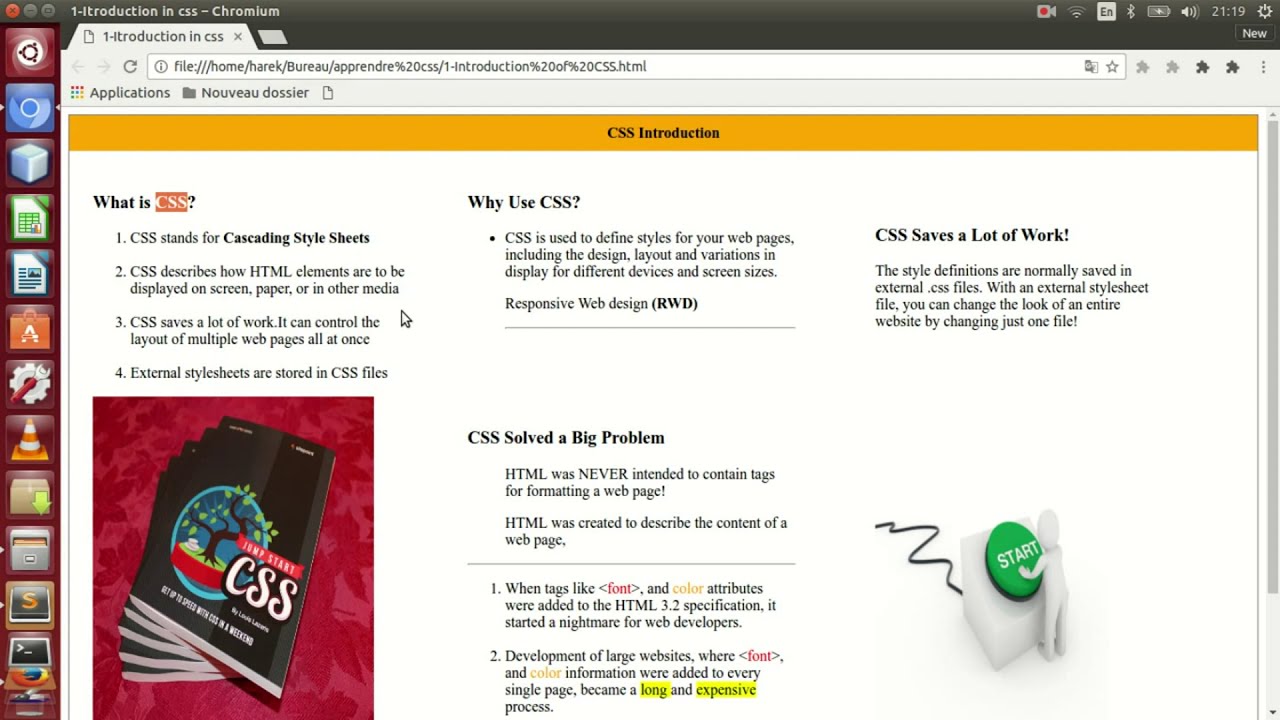The image is a screenshot of a computer's graphical user interface, likely from a Mac or a Linux operating system, featuring a web browser labeled "CSS-Chromium." The browser displays a basic HTML web page dedicated to an "Introduction to CSS" course, albeit with a misspelling as "Itroduction." The layout includes a horizontal menu bar at the top and a left side menu bar with various application icons. The main content area, with a white background, is divided into several blocks of black text discussing topics like "What is CSS?", "Why use CSS?", "CSS solved a big problem," and "CSS saves a lot of work." These sections contain bullet points and lists elaborating on the respective topics. The bottom left corner of the page features an image of a stack of CSS textbooks placed on a floor, while the bottom right includes a 3D illustration of a small man pressing a large green button labeled "Start." Overall, the detailed and structured interface conveys an organized approach to learning CSS.